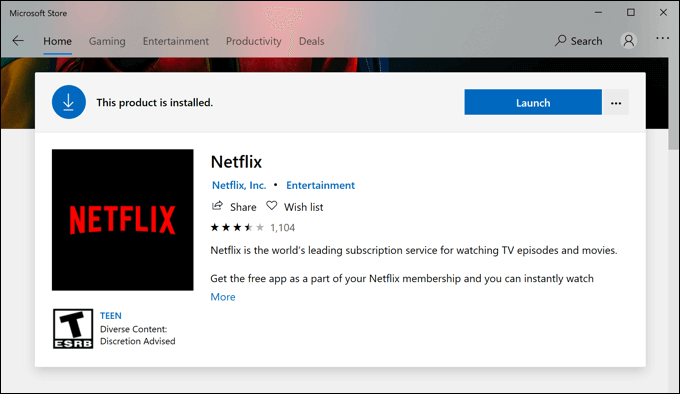Displayed here is a detailed shot from the Microsoft Store. On the right side of the screen is the search bar. In the center of the screen, a pop-up indicates that the product is already installed with the option to "Launch" it. The product in question is the Netflix app, developed by Netflix, Inc.

Netflix is described as the world's leading subscription service for watching TV episodes and movies. The text encourages users to get the free app as part of their Netflix membership for instant streaming of content. For more details, users are prompted to click "More."

Below the Netflix logo, there is an ESRB rating in a square box showing a "T" for Teen, indicating diverse content with a recommendation for viewer discretion.